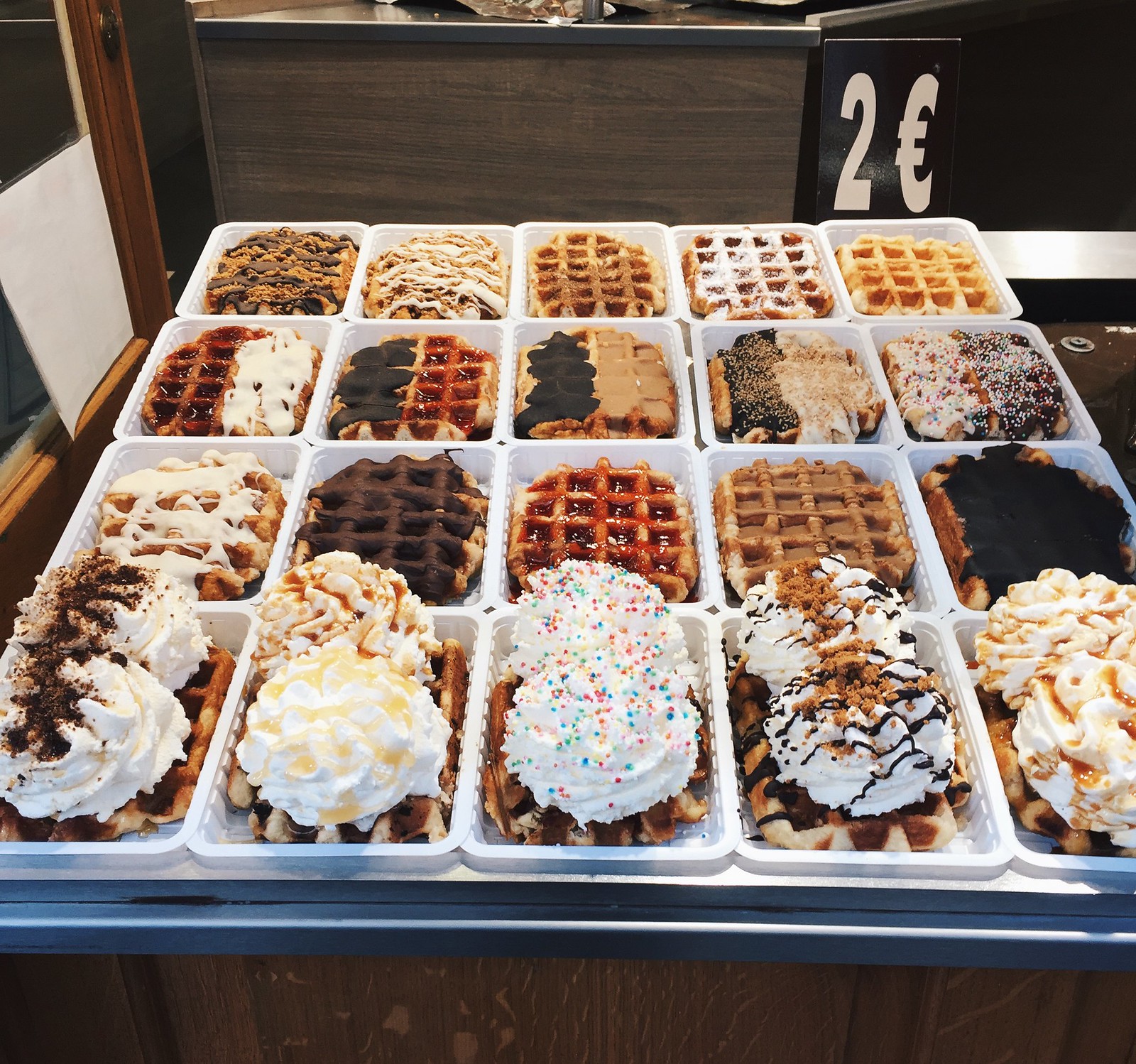The image captures an ornate wooden pastry cabinet within what appears to be a bakery. Inside the case, a white sectioned tray meticulously organizes 20 waffles into four rows of five, each progressively more decadent from top to bottom. The top row features relatively plain waffles, adorned with simple toppings like confectioner's sugar and maple syrup. As your gaze moves downwards, the waffles become increasingly embellished, starting with two-tone frosting and cream, transitioning to whipped cream crowned with various garnishes including colored sprinkles, cinnamon, coconut, and intricate chocolate swirls. The bottom row showcases waffles topped with ice cream swirls and even more elaborate decorations, like butterscotch and caramel drizzles.

Each waffle in the display offers a unique visual treat. The front row of waffles is garnished with whipped cream, adorned with toppings such as chocolate sprinkles, caramel drizzle, and cookie crumbs. Subsequent rows feature combinations of crunchy chocolate, strawberry sauce, and powdered sugar, as well as half-and-half designs that mix different toppings on each waffle. A conspicuous black sign in the backdrop reads “two euros,” indicating the price.

The entire display is a feast for the eyes, not just for its vibrant assortment of waffles but also for the intricate details and varying toppings that make each waffle distinct and sumptuous.